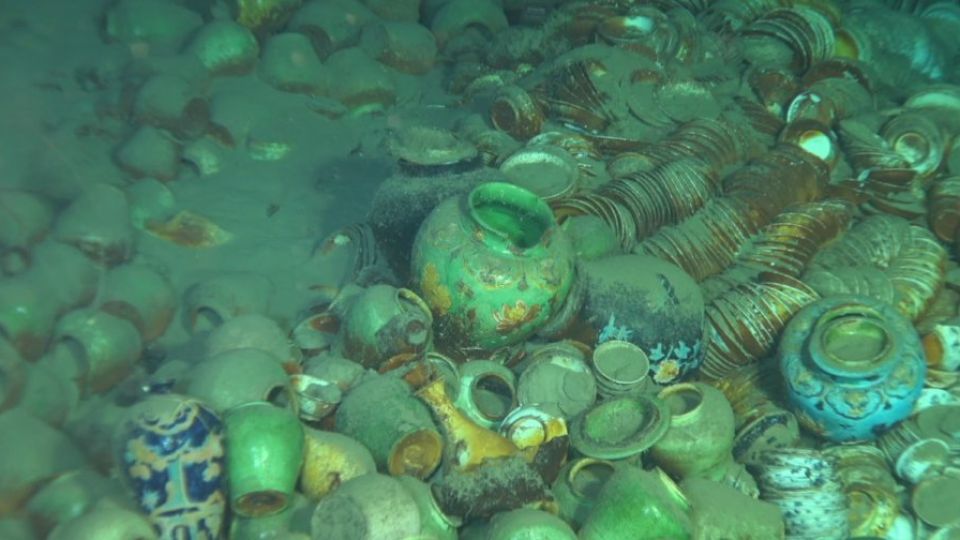This photograph captures an underwater scene of the sea floor densely scattered with various types of pottery, including clay pots, ceramic pots, and metal vessels, some of which appear corroded. The predominant hues are a blend of light green, pale blue, and bronze tones, suggesting a layer of tarnish and sand covering many of the items. In the foreground, notable pieces include a bright blue pot, a dark blue pot with a yellowish pattern, and a light blue pot. Additionally, a large vessel with a bronzed copper color and hints of green sits prominently at the center. Some pots are even stacked, creating a layered effect that extends into the background, where hundreds of bronze-toned pottery pieces can be seen interspersed with sand. The overall impression is that of a historical underwater trove, with decorative elements partially obscured and a distinctive blue-green patina enveloping the scene.